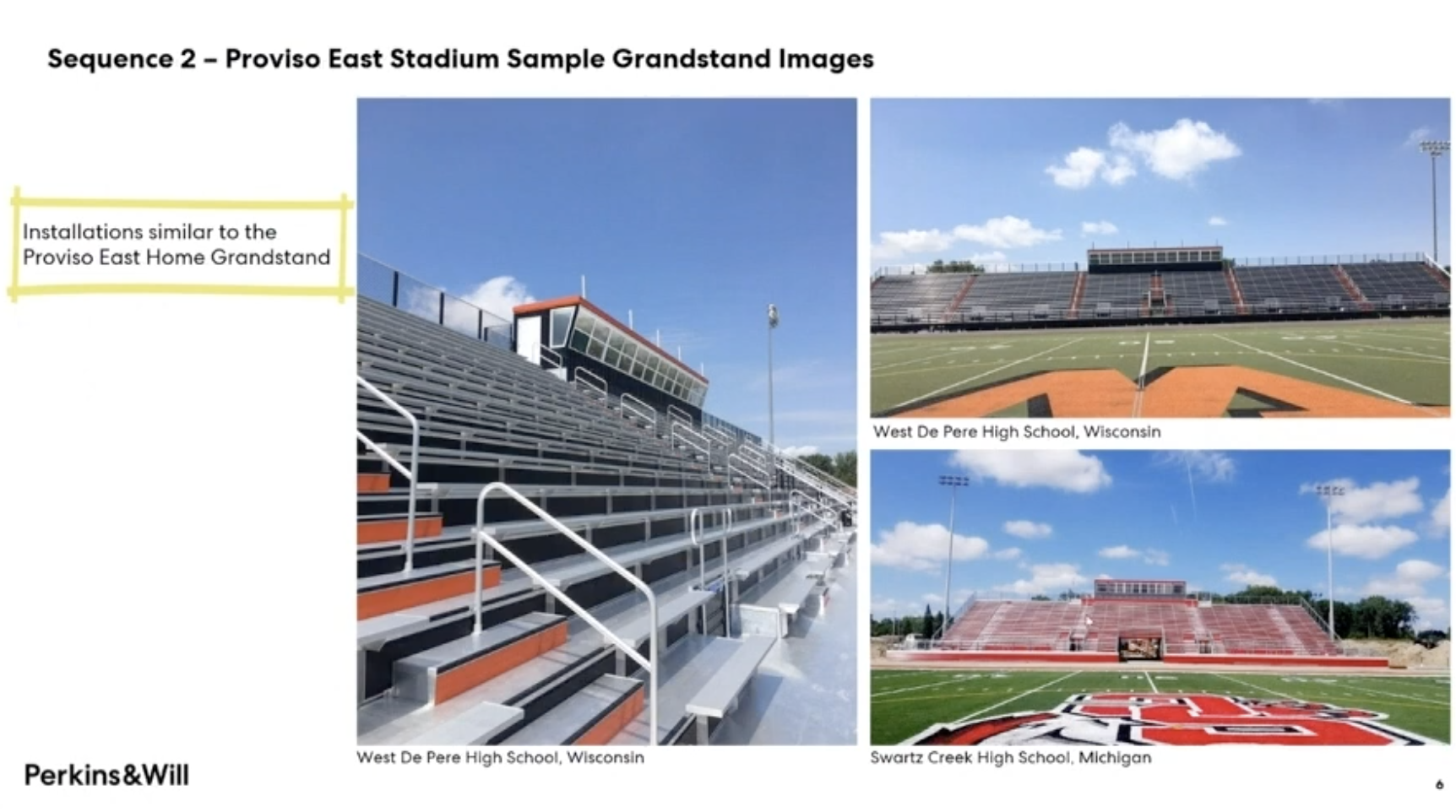The image consists of three different photographs of football stadiums, likely part of a company's portfolio showcasing past installations. In the top left corner, a black bold title reads, "Sequence 2 - Proviso East Stadium Sample Grandstand Images." Below this heading, a yellow rectangle contains the text, "Installation Similar to the Proviso East Home Grandstand," also in black. The three stadium photographs are arranged with the first photo on the left side, showing bleachers and an enclosed announcer's platform, labeled below as "West D. Perry High School, Wisconsin." The second photo, situated in the upper right, features a field-level view with orange elements, also labeled "West D. Perry High School, Wisconsin." The third photo, positioned in the lower right, displays a stadium with red highlights and a field logo, labeled "Swartz Creek High School, Michigan." At the bottom left corner of the image, the black text "Perkins and Will" appears, suggesting it’s the logo or brand responsible for these installations. The entire presentation is set against a white background.